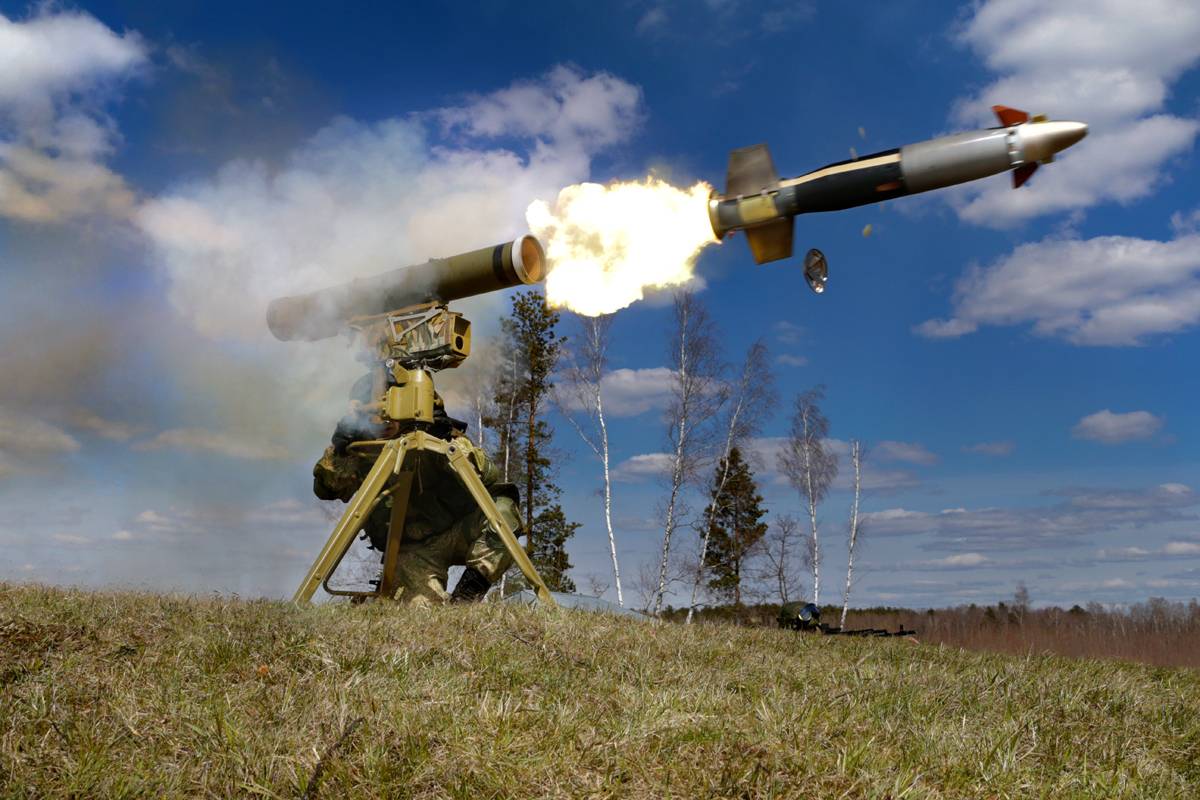The photograph captures a highly detailed and intense scene of a wartime practice or live military exercise, focusing on a soldier positioned centrally and kneeling on both knees in a camouflage uniform. The soldier is operating a three-legged missile launcher, which dominates the frame. The missile is captured mid-launch, bursting out of the launcher tube with vivid flames and smoke trailing behind it. The backdrop features a mix of dead or dying grass in the foreground, with dense, green trees and a partly cloudy sky, indicating it's daytime. This powerful image showcases the precise moment of a missile being fired, combining dramatic natural elements with the striking force of military technology.